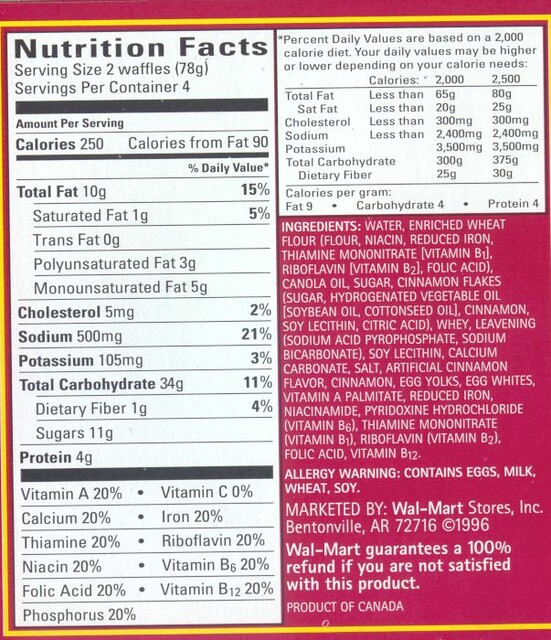The image showcases a detailed Nutrition Facts label for a food product, specifically waffles, from Walmart. The label is predominantly white, set against a dark pink background with a yellow outline. At the top, it specifies the serving size as two waffles, with four servings per container. Key nutritional information includes 250 calories per serving, 90 of which are from fat. The label is organized into a chart-style format, detailing total fat, saturated fat, trans fat, and other nutritional values. The ingredients list is extensive, including enriched wheat flour, niacin, reduced iron, thiamine mononitrate (vitamin B1), canola oil, sugar, cinnamon flakes, soy lecithin, calcium carbonate, salt, artificial cinnamon flavor, and both egg yolks and egg whites. There is also an allergy warning indicating the presence of eggs, milk, wheat, and soy. Additionally, the label notes that the product is marketed by Walmart Stores, Inc. in Bentonville, Arkansas, and offers a guarantee of a 100% refund if not satisfied. The product is identified as a product of Canada. The percent daily values are based on a 2,000 calorie diet.